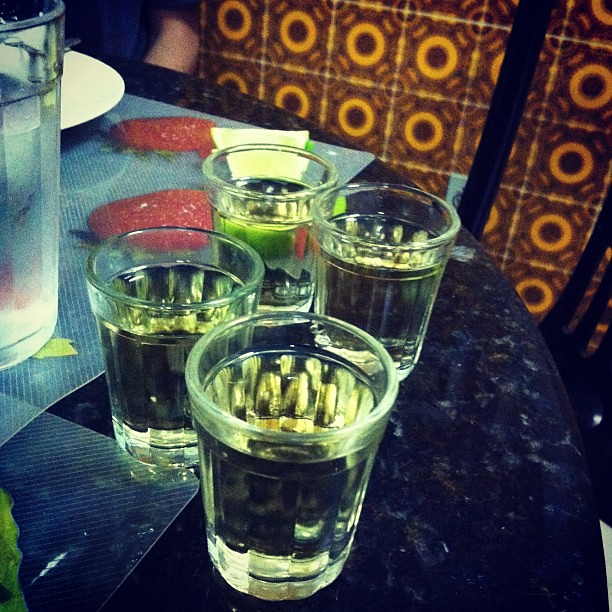The image depicts a detailed setting on a dark blue marble-surfaced table adorned with a light blue tablecloth. At the center of the table are four shot glasses filled nearly to the brim with a clear liquid, likely water, arranged in a precise diamond pattern. To the left of the shot glasses sits a white plate, and a pitcher of water, along with two small, unidentified pink objects. The table also features clear plastic placemats, possibly decorated with red strawberries or fruits, adding a subtle touch of color. In the background, the top left corner partially shows an elbow, hinting at a person's presence. The backdrop consists of a maroon and gold mosaic-designed wall with distinctive yellow circles, adding a rich, ornate feel to the scene. There also appears to be a chair or object adorned with a brown, circular, and block pattern, peeking from behind the table.